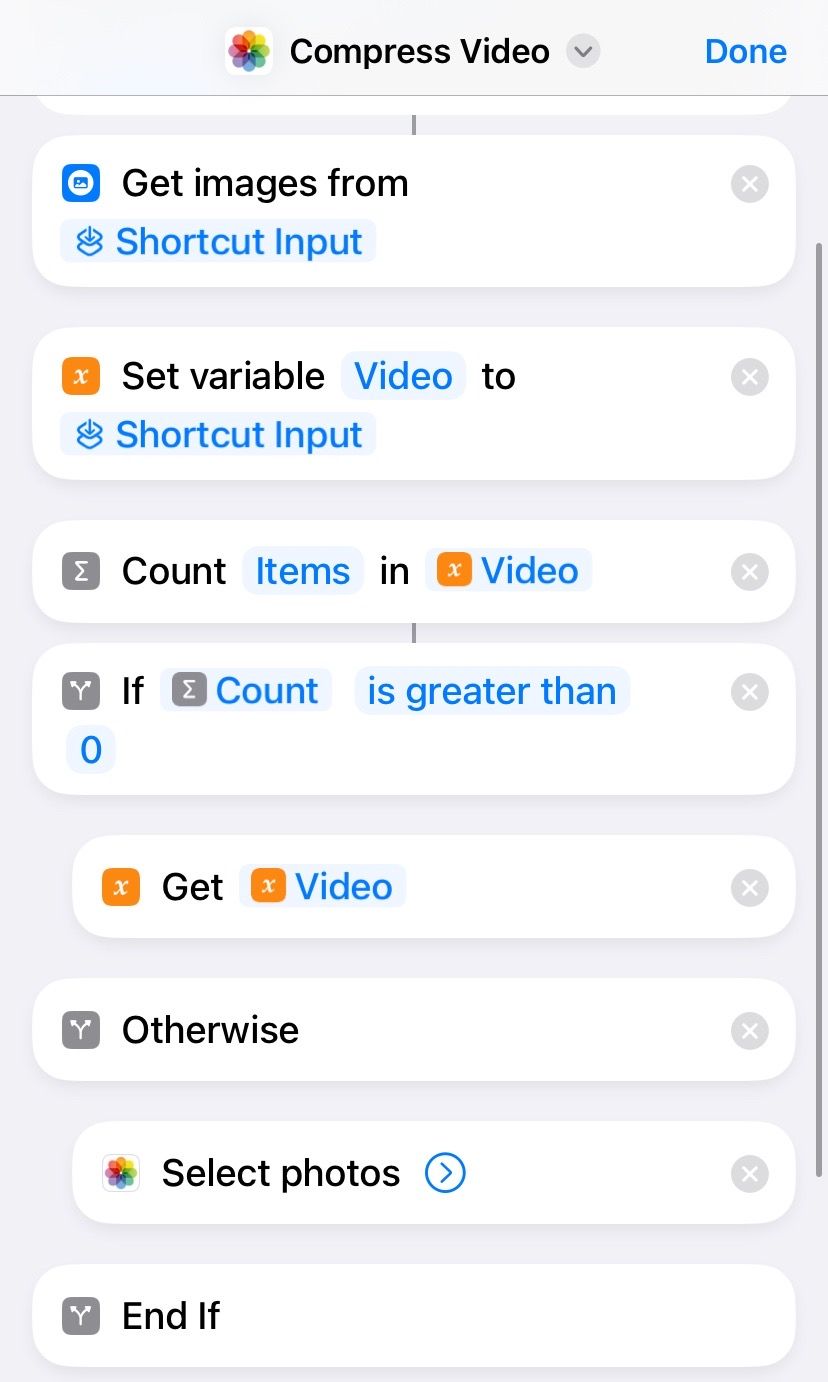This image is a screenshot from an iPhone, specifically from within the Photos application as indicated by the light gray header at the top and the distinctive Photos icon, represented by the traditional flower, positioned to the left of the title. The centered title reads "Compress Video" in bold black font. To the right of this title, there is a circular icon in light gray featuring a dark gray arrowhead pointing downwards, followed by a blue "Done" text in bold.

Beneath this header, a thin gray border demarcates the top portion of the interface from the main content area, which consists of several sections designed in rounded rectangles with white backgrounds. The first section reads "Get images from" in black text, followed by a highlighted light blue area with bold bright blue text "Shortcut Input." In the top right corner of this section is a light gray circle containing a white 'X'.

The next section, also a rounded rectangle, is labeled "Set variable" in black text. Within a light blue highlighted area, bold blue text reads "Video," followed by black text saying "to," and then another light blue highlighted text "Shortcut Input." This section, too, has a small light gray circle with a white 'X' in the top right corner.

Following this, a smaller rectangular area labeled "Count" in black text appears. It includes a highlighted area indicating "Items," followed by black text "in," and then another highlighted text "Video." An orange square icon is positioned to the left of the highlighted "Video" text.